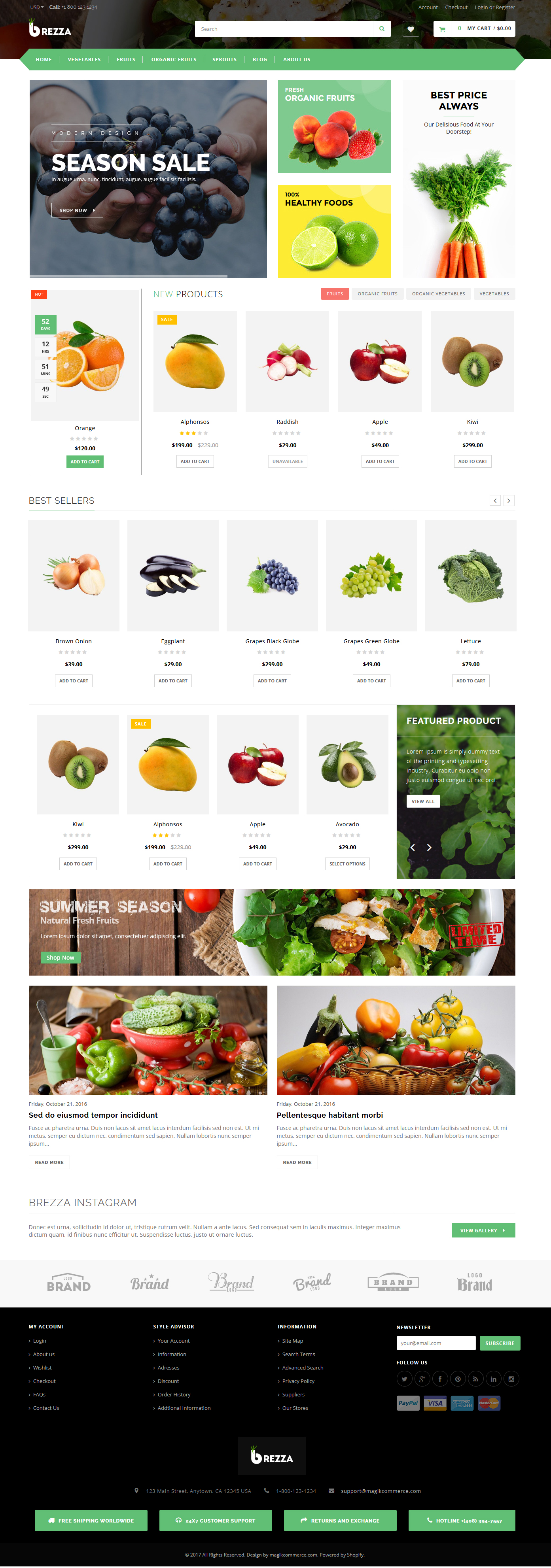This is a detailed screenshot of a website featuring a variety of fruits and vegetables. The overall layout is intricate with numerous small and nearly unreadable text elements. At the top of the image is a black background containing a white box. Below this is a green bar featuring some white text. Prominently displayed is a photograph of two hands holding a bunch of blueberries, overlaid with the text "Season Sale" in white.

The page showcases multiple vibrant images of fresh produce. There is a clear and detailed picture of a green lime, halved to display its juicy interior. Adjacent to it is an image of several carrots, complete with bushy green tops. The citrus section includes a vivid photograph of oranges, featuring one whole orange, a halved orange, and a single orange slice. 

Nearby, a yellow lemon with a green leaf stands out, followed by an image of apples showing two whole apples and one cut in half. The exotic kiwi is also present, with two whole kiwis and one sliced open to reveal its delicious green flesh.

Grapes are featured in abundance with separate pictures of green and purple varieties. There is also a detailed photo showcasing two whole onions and one halved onion. Complementing these are images of a salad with the caption "Summer Season" written in bold white text, and a vibrant picture containing both a green pepper and an orange pepper.

Overall, the screenshot captures a colorful and diverse collection of fresh produce, emphasizing the seasonal theme and visually appealing to viewers.